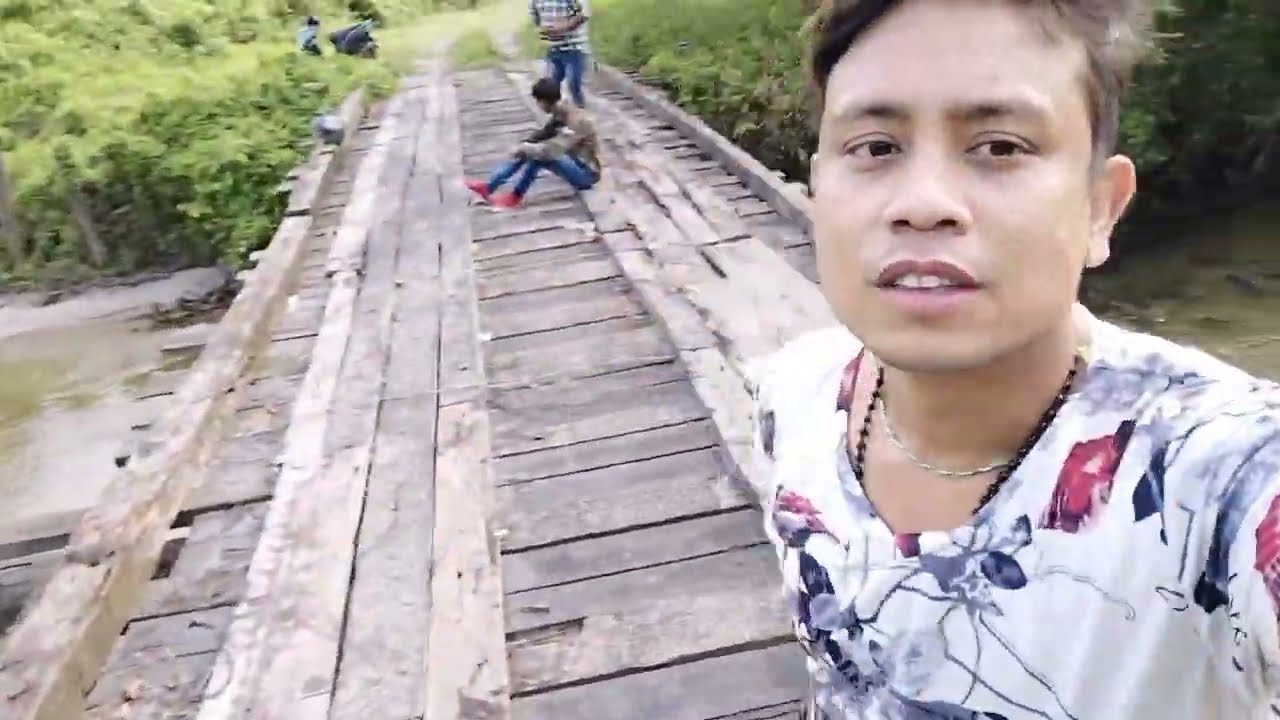This color photograph captures a young man taking a selfie on an old wooden bridge. Positioned on the right side of the image, he is wearing a distinctive white shirt adorned with a floral and bird design in shades of red, black, and perhaps blue. Around his neck hang a black beaded necklace and a silver one. The man’s left arm is extended, holding the camera, and his gaze is directed to the left of the lens.

Behind him, the weathered wooden bridge stretches across a murky, greenish-brown river, surrounded by lush greenery including small shrubs and bushes. On the bridge, two other men in jeans and shirts are visible: one wears red shoes and is sitting, while the other stands nearby. Additionally, a motorcycle or scooter can be seen parked at the far end of the bridge, from which a dirt road leads off into the distance, enhancing the rural, outdoor setting. In the background, more people are visible amidst the green foliage, contributing to the overall scene of a peaceful, rustic environment.